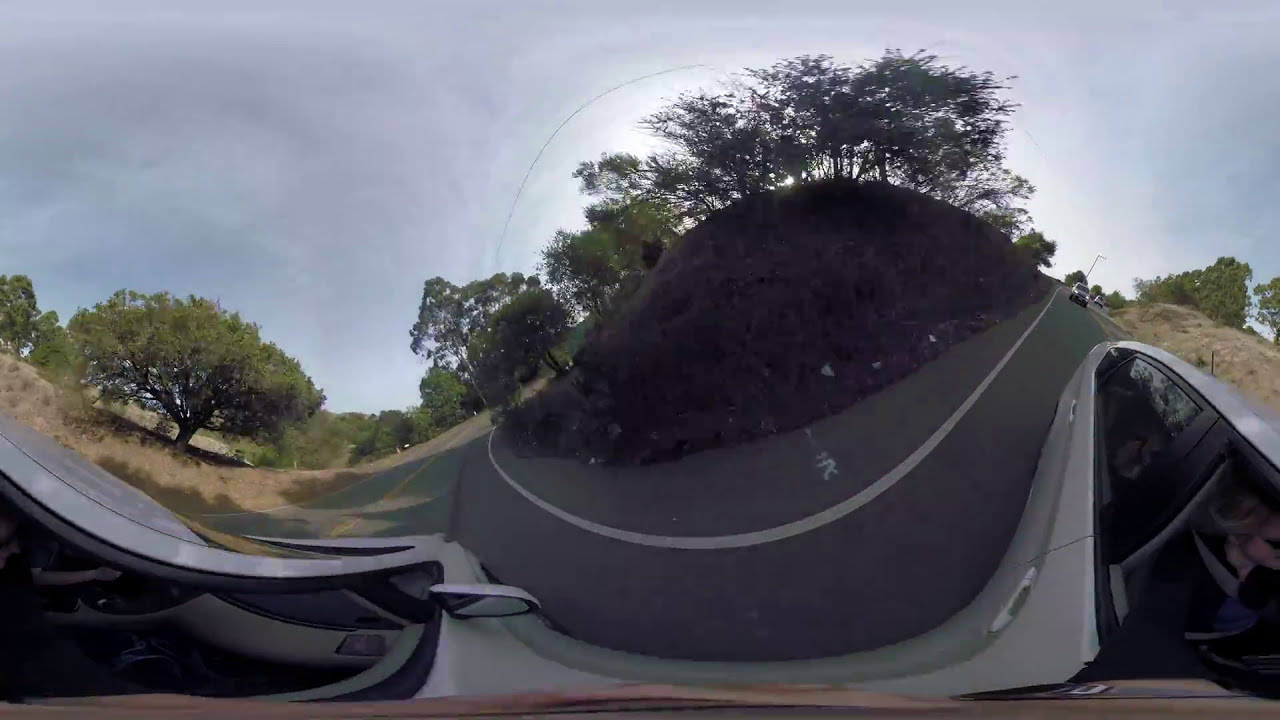This highly distorted and warped wide-angle photo, likely taken using a VR or 360-degree camera, captures the perspective from inside a white vehicle. The image wraps around with a 180-degree view, showing parts of the car on the right side, curving underneath to the left side. The road also curves around a central dirt hill topped with several trees, adding to the surreal appearance. Scattered trees and bushes are visible in the background, with a notable large tree on the left. The photo features a cloudy sky and a field of yellow grass on the left side, enhancing the outdoor scene. Behind the visible car, one can see additional vehicles trailing, indicating traffic. The visual experience is further intensified by the warped effect, making the car appear as if it dips and arches across the frame from left to right. Yellow road lines and a mix of greenery complete this uniquely captured landscape.